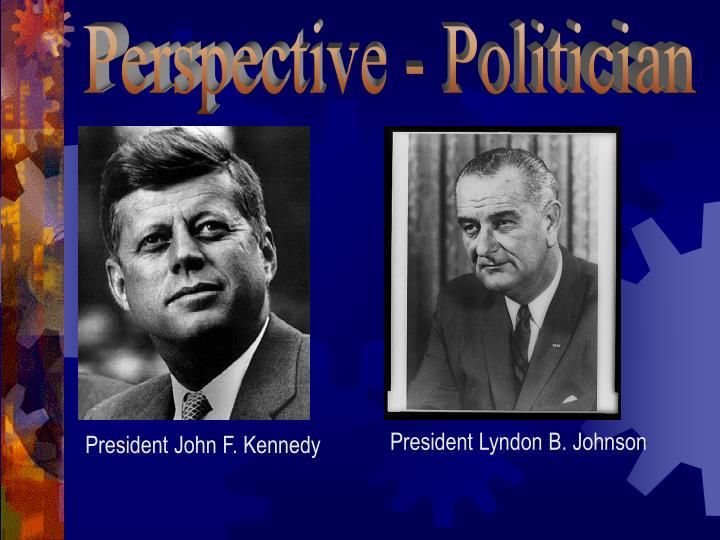The image features a vivid blue background adorned with silhouettes of gears in various blue tones. Towards the left side, a narrow vertical band displays additional gear silhouettes in shades of red, blue, and gray. Dominating the top of the composition is the text "Perspective-Politician" in orange-ish letters with a drop shadow effect, creating a prominent header. Below this, two black-and-white photographs are prominently placed: on the left is John F. Kennedy with the caption "President John F. Kennedy" in white lettering, and on the right is Lyndon B. Johnson with the caption "President Lyndon B. Johnson" in white lettering. The entire image gives an impression of a well-designed visual, potentially a PowerPoint slide, incorporating elements of political history and mechanical designs to create a striking and informative visual presentation.